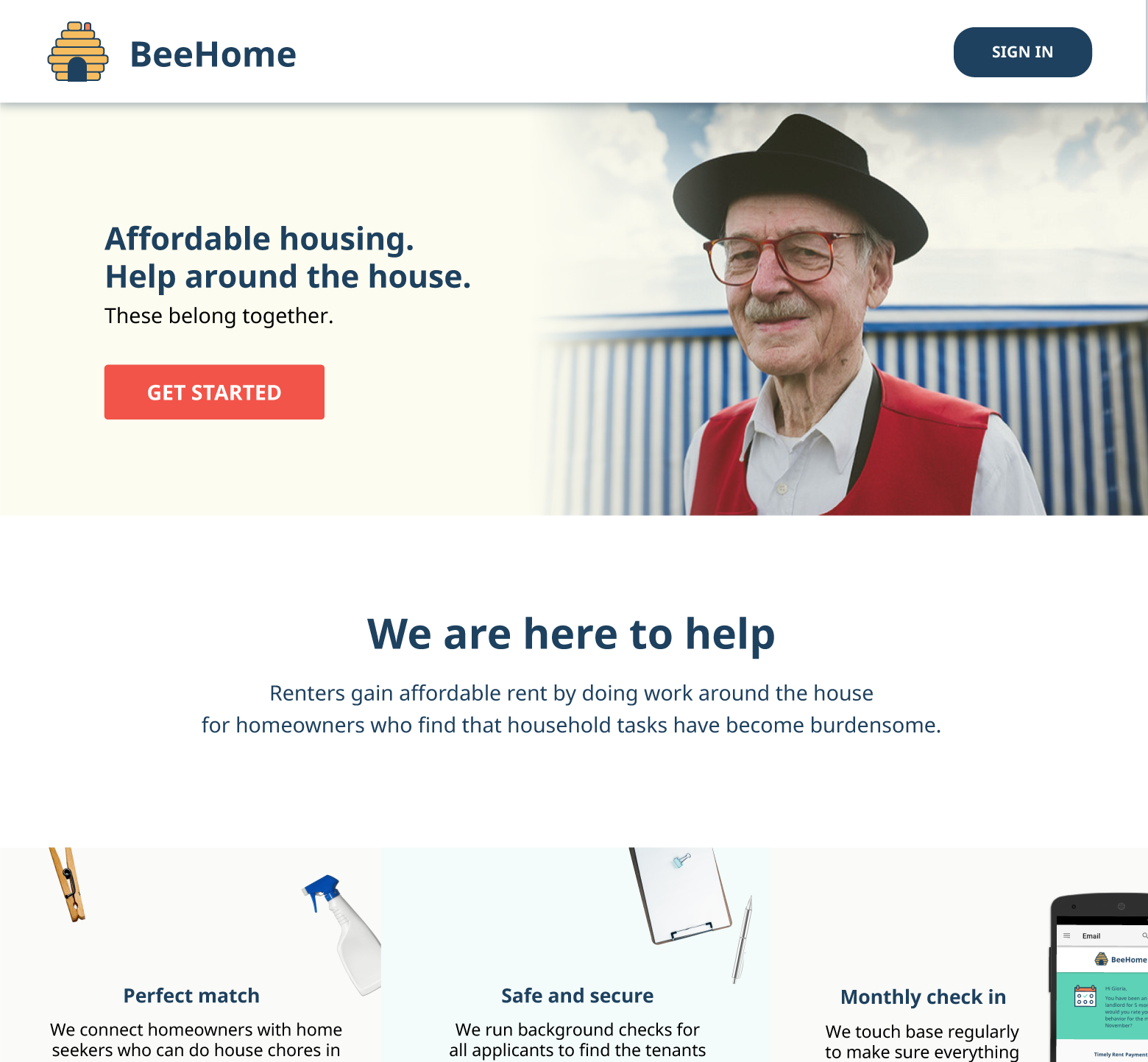The image features a logo resembling a geometric bee nest, followed by the text "Bee Home." Next to it is a black sign-in button. Below this, there's a description that reads, "Affordable housing. Help around the house. These belong together." A prominent red box labeled "Get Started" is also displayed.

On the right side of the image, there is a picture of an elderly man wearing a black wide-brim hat, glasses, a mustache, a white collared shirt, and a red vest. Below this image, text reads, "We're here to help renters gain affordable rent by doing work around the house for homeowners who find household tasks have become burdensome."

Further down, the text continues, "Perfect match: We connect homeowners with home seekers who can do the house chores," accompanied by icons of a clothespin and a spray bottle. The tagline "Safe and secure: We run background checks for all applicants to find a tenant," is also present. The image concludes with "Monthly check-in: We touch base regularly to make sure everything is going smoothly."